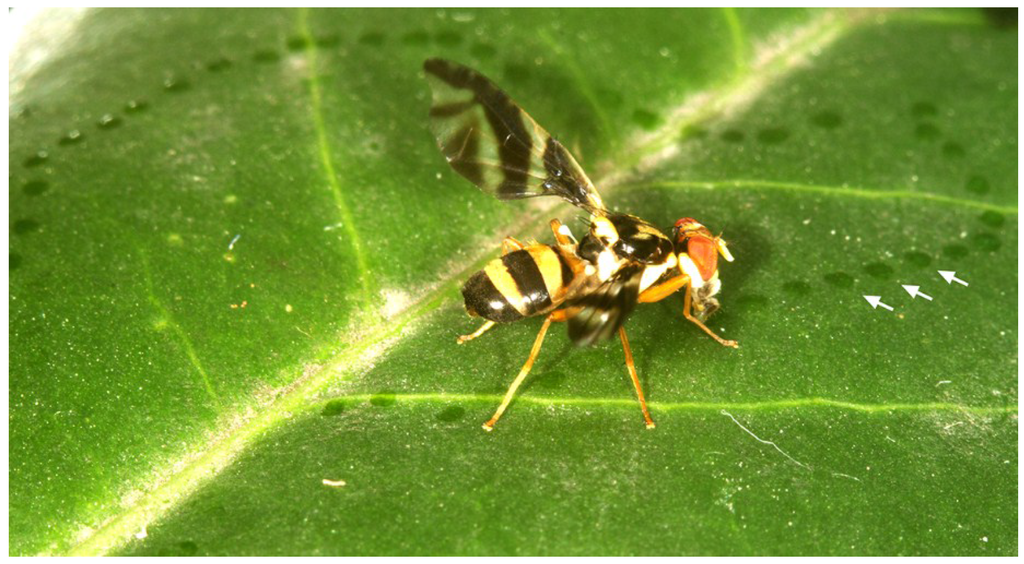This close-up photograph captures a striking image of a black and yellow striped wasp resting on a vividly green leaf. The wasp, easily mistaken for a bee, has its six legs firmly planted on the leaf while its wings are spread apart, revealing black stripes on its translucent surfaces. The insect's abdomen showcases distinct black and yellow banding, and its pronounced yellow eyes and formidable mandibles add to its detailed appearance.

The leaf beneath the wasp features a prominent white vein running through the center, with multiple smaller veins branching out to the sides. Upon closer inspection, one can observe a series of nearly perfect round dots or small circular wet spots dotting the surface of the leaf, almost like a trail left by the wasp. There are three white arrows superimposed on the photograph, each indicating these round dots. The arrows point to the left, drawing attention to the peculiar trail that contrasts with the leaf's otherwise clean surface. This fascinating detail hints at the wasp's interaction with its environment, adding an element of curiosity to the image.